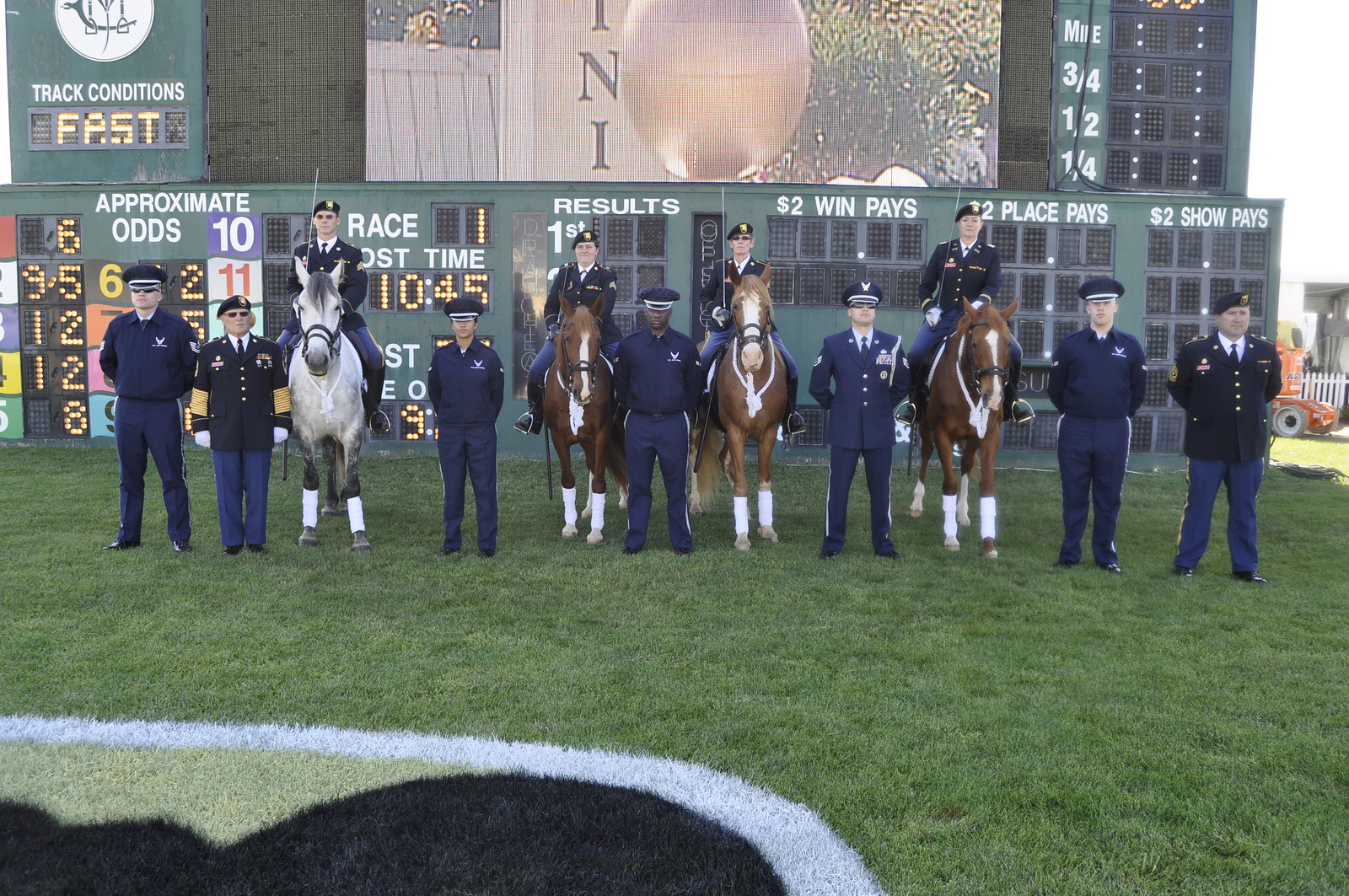This image captures a group of military officers and personnel, totaling 14 men, standing in front of a racetrack scoreboard. The scoreboard, painted green with white text and yellow digital displays, features race times, results, and odds. The men are dressed in navy blue uniforms, comprising jackets and blue pants, with some donning windbreaker jackets paired with blue pants adorned with a white stripe. The group is arranged with four officers mounted on horses, which are positioned alternately with standing personnel. The horses, three of which are brown with white streaks down their muzzles, white chests, and white stockings up to their knees, and one gray horse with black legs, add an equestrian element to the scene. All individuals are staring directly at the camera, standing on a field of lush green grass. The meticulous placement, uniform attire, and the racetrack ambiance create a detailed and structured composition in this photograph.